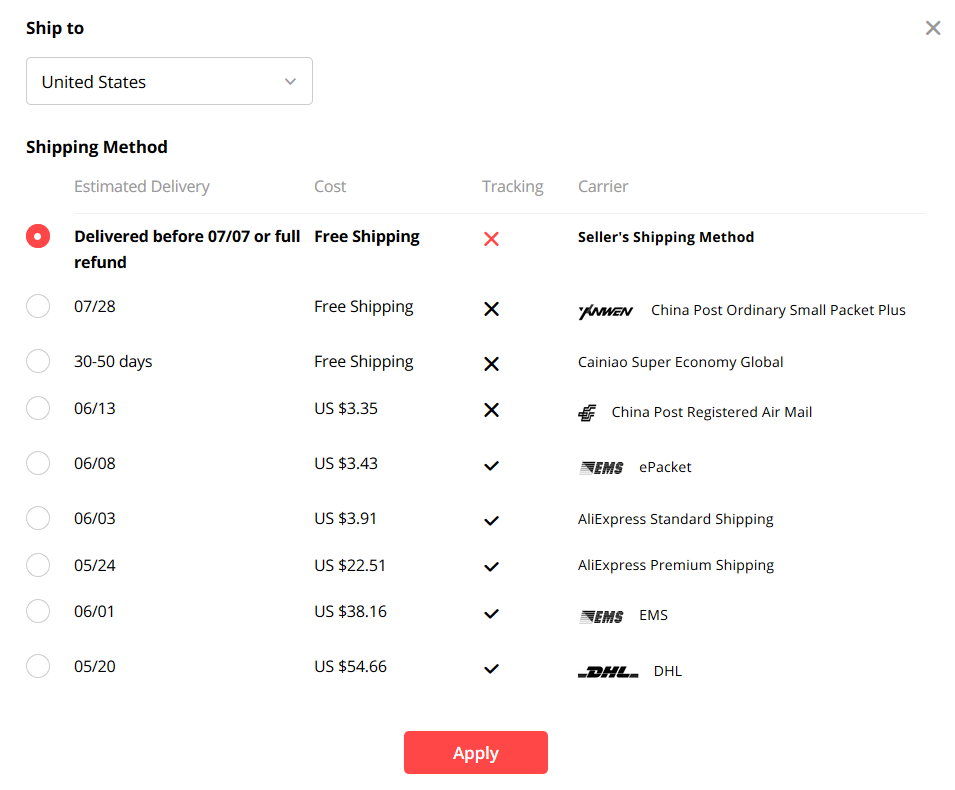This screenshot captures the shipping information section on an e-commerce website. The interface features a clean white background. 

**Top Left:**
- The bold header "Ship To" is prominently displayed. Below, a drop-down menu shows the selected country as "United States" with an arrow indicating additional options.

**Top Right:**
- A medium gray "X" icon is present, likely for closing the shipping information modal or section.

**Below the Drop-down Menu:**
- A bold text heading reads "Shipping Method." This is followed by labels for four columns: "Estimated Delivery," "Cost," "Tracking," and "Carrier," all written in light gray text.

**Shipping Options:**
- There are several shipping options listed, each accompanied by a radio button. 

1. **First Option (Selected):**
   - Contains a red-dotted (donut-style) selection indicator.
   - **Text (bolded)**:
     - **Estimated Delivery:** Delivered Before 07-07 or Full Refund
     - **Cost:** Free Shipping
     - **Tracking:** Red "X" (indicating no tracking available)
     - **Carrier:** Seller's Shipping Method
   
2. **Second Option:**
   - Contains an unselected white radio button.
   - **Text:**
     - **Estimated Delivery:** 07-28
     - **Cost:** Free Shipping
     - **Tracking:** No Tracking
     - **Carrier:** [Anwen Logo], China Post Ordinary Small Packet Plus

3. **Third Option:**
   - Contains an unselected white radio button.
   - **Text:**
     - **Estimated Delivery:** 30-50 Days
     - **Cost:** Free Shipping
     - **Tracking:** No Tracking
     - **Carrier:** Kai Niao, Super Economy Global

4. **Fourth Option:**
   - Contains an unselected white radio button.
   - **Text:**
     - **Estimated Delivery:** 06-13
     - **Cost:** US $3.35
     - **Tracking:** No Tracking
     - **Carrier:** China Post Registered Air Mail

5. **Fifth Option:**
   - Contains an unselected white radio button.
   - **Text:**
     - **Estimated Delivery:** 06-08
     - **Cost:** US $3.43
     - **Tracking:** Includes Tracking
     - **Carrier:** ePacket

**Additional Options:**
- There are four more shipping options listed below, but their details are not captured in this description.

Everything is neatly organized, making it easy for users to compare and choose the most suitable shipping method based on delivery time, cost, tracking availability, and carrier service.